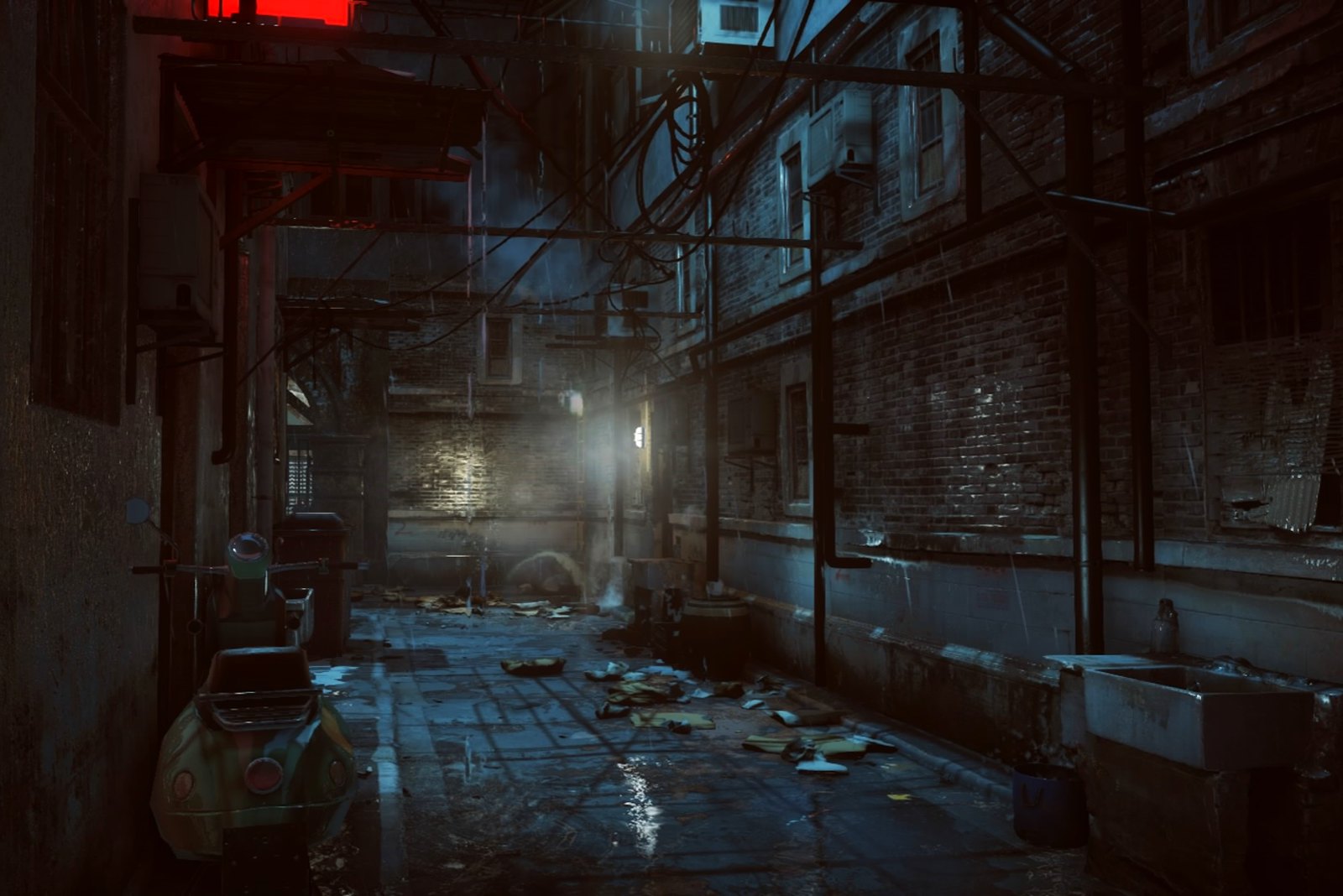The image depicts a narrow, dimly lit alleyway typical of those found in large urban areas. The alley's surface is composed of stone with a gray hue, interspersed with darker colored masonry. The ground is strewn with debris, including discarded boxes and light-colored packaging, contributing to a general sense of untidiness. Flanked by tall buildings on either side, the alley extends to a junction where it appears to open up, offering pathways to both the left and right. The buildings, constructed predominantly of brick and stone, feature steel frameworks likely intended for fire escapes. These structures extend upwards beyond the frame of the image, indicating their considerable height. On the left side, just out of full view, the bottom portion of a red neon sign can be seen, adding a touch of vivid color to the otherwise muted scene.